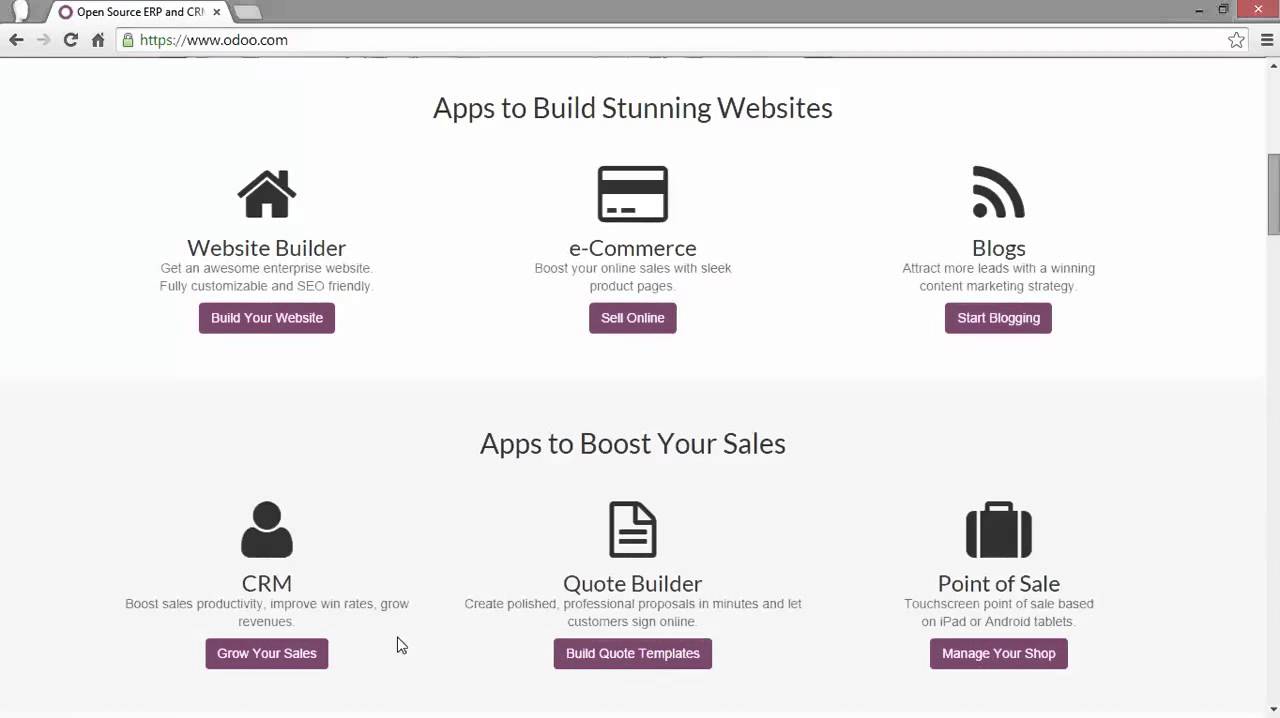This screenshot features an open web page from the Odoo website, as noted in the browser's address bar (https://www.odoo.com). The page is an overview of various applications offered by Odoo to enhance business operations.

At the top center of the webpage, there's a section titled "Apps to Build Stunning Websites." In this section, three primary apps are listed from left to right:
1. **Website Builder**: Promises to deliver an awesome enterprise website that is fully customizable and SEO-friendly.
2. **E-commerce**: Aims to boost online sales with sleek product pages.
3. **Blogs**: Designed to attract more leads through a compelling content marketing strategy.

Below this, there is another section titled "Apps to Boost Your Sales." Within it, two key apps are highlighted:
1. **CRM**: Focused on boosting sales productivity, improving win rates, and growing revenues. Beneath this description is a prominent purple action button labeled "Grow Your Sales."
2. **Quote Builder**: Offers tools to create polished, professional proposals in minutes and allows customers to sign them online. Below this description is another purple action button labeled "Build Quote Templates."

The layout emphasizes ease of navigation and the strategic benefit each app offers, visually organized to guide users towards action.